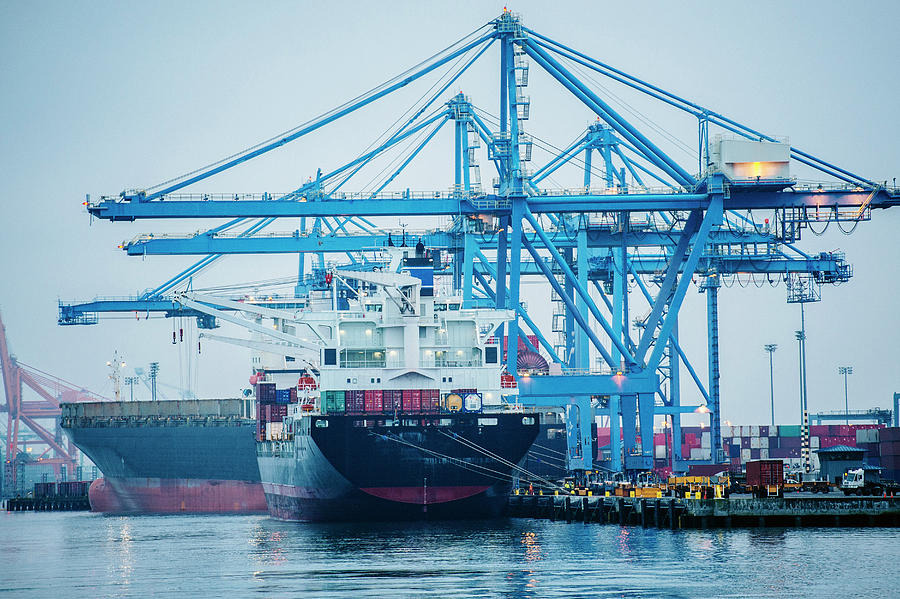This outdoor photo captures a bustling port scene during an overcast day, where the sky is a solid gray, casting a bluish hue over the entire image. In the foreground, there is a large cargo ship facing the photographer, with its hull painted blue at the top and red at the bottom. The ship is loaded with multicolored cargo containers, including yellow, red, and other vibrant hues. Surrounding the vessel are three massive blue cranes actively loading and unloading containers. These towering cranes dominate the landscape and are essential to the port's operations. Behind the primary ship, another cargo vessel is parked horizontally, also featuring a blue and red hull. The second ship is parallel to the dockline, contrasting the orientation of the front-facing ship. At the bottom of the image, we see the reflective surface of the water, while the port itself is busy with vehicles, trucks, and stacks of cargo containers piled high. This detailed scene epitomizes the industrious atmosphere of modern maritime logistics.